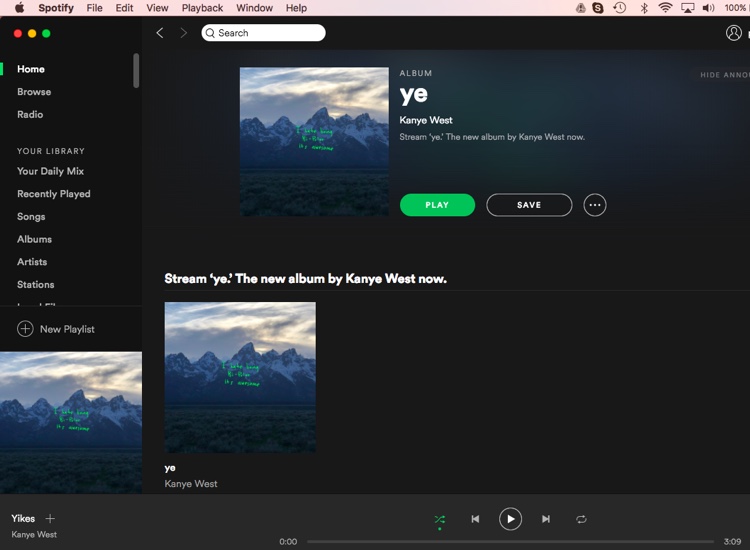The screenshot captures the Spotify application running on a macOS device. The top border of the screen features a light pink background combined with standard macOS system icons and options. Specifically, from left to right, there is an Apple logo followed by menu items: Spotify, File, Edit, View, Playback, Window, and Help. Additionally, several system icons are visible: a Skype logo, a stopwatch icon, a Bluetooth icon, and icons representing Wi-Fi connectivity and volume control.

Beneath the menu bar, there is a Spotify interface with a search bar labeled “Window.” The left-hand sidebar of the interface displays various navigation options, which include: Home, Browse, Radio, Your Library, Your Daily Mix, Recently Played, Songs, Albums, Artists, and Stations.

Prominently displayed is a promotional banner for Kanye West's new album "Ye." This banner appears in three locations: twice on the right side and once towards the upper center of the screen. The banner features an image of mountains under a cloudy sky, suggesting an early morning scene with low light conditions. Accompanying the image is the text "Stream Ye, the new album by Kanye West now," along with two buttons: a green play button for streaming the album and a black save button for adding it to the user's library.